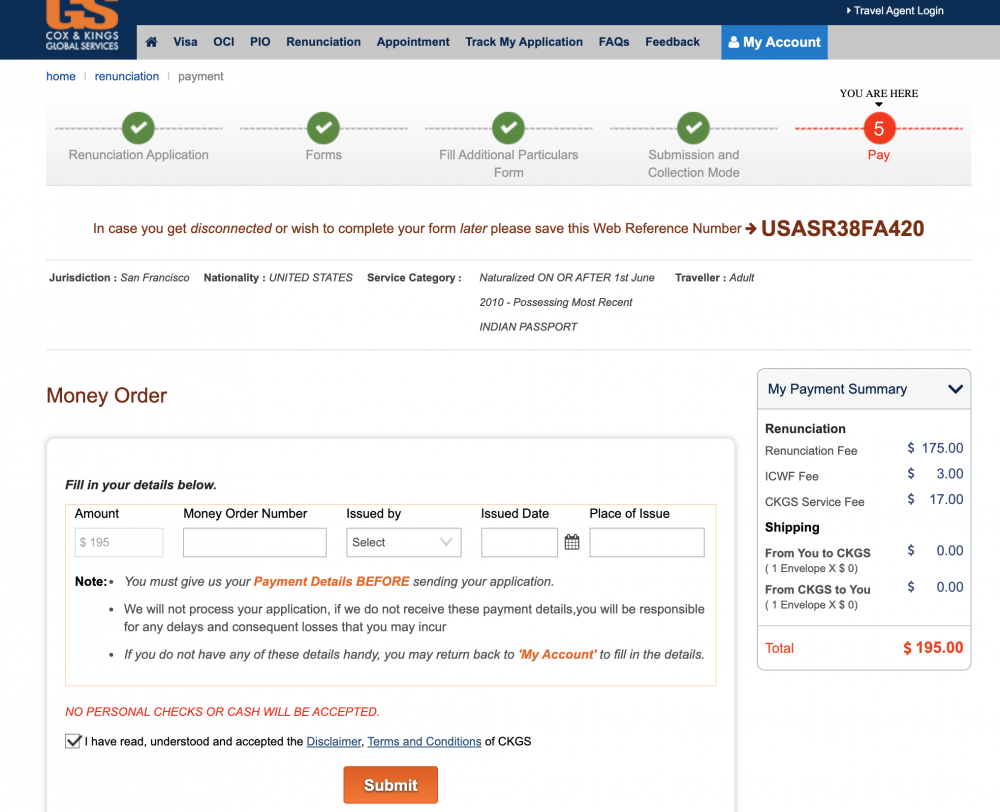Title: Detailed Breakdown of Cox and King's Global Services Payment Form

Caption: 

At the top of the form, there are prominent orange letters "G" and "S" followed by "Cox and King's Global Services." Beneath this, there are three green circles with white check marks, each denoting different steps: "Reunification Application," "Fill Additional Particulars Form," and "Submission and Collection Mode." 

To the far right, a red circle with the number "5" inside indicates the current step, labeled "Pay," with a notation above it stating "You are here." 

Moving downward, there is a section titled "Money Order" that instructs to "Fill in your details below." The required fields include:
- **Amount:** $195
- **Money Order Number:** [Empty Box]
- **Issued By:** [Empty Box]
- **Issued Date:** [Empty Box]
- **Place of Issue:** [Empty Box]

To the right, within a vertical square labeled "My Payment Summary," the fees are itemized as follows:
- Reunification Fee: $175
- ICWF Fee: $3
- CKGS Service Fee: $17
- Shipping from you to CKGS: $0

The total amount due is emphasized in red text with a red dollar sign indicating the sum of $195.